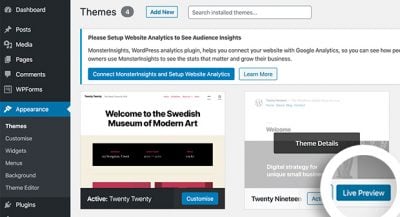In this vertical image, we see a user interface divided into two primary sections. On the left side, which features a black background, there is a vertical menu starting from the top with the following options: "Dashboard," "Posts," "Media," "Pages," "Comments," "Wi-Fi," "Forms," "Appearance," and "Themes." The menu continues with five additional items that are blurred and illegible.

On the right side, the top of the page prominently displays the word "Themes" in black text. Below this heading, there is a button labeled "Add New" and a search bar. Following the search bar, there is a message stating, "Please set up website analytics to see Analytics insights." 

Underneath this message, several lines of text appear, but they are not fully legible. There is a noticeable blue box featuring the word "Connect," accompanied by another unreadable element. Beside this, a "Learn More" button is situated.

Lower down in this section, there are two image previews. The image on the left welcomes viewers to the "Swedish Museum of Modern Art" and includes a black rectangular button along with two smaller pink buttons below it. It also mentions "Active 2020" and a blue button that appears to say "Questions."

To the right is an image with a white background, highlighting a central gray box. Above this gray box, a black box contains the text "Theme Details." In the bottom right corner of this image, a blue button is labeled "Live Preview."